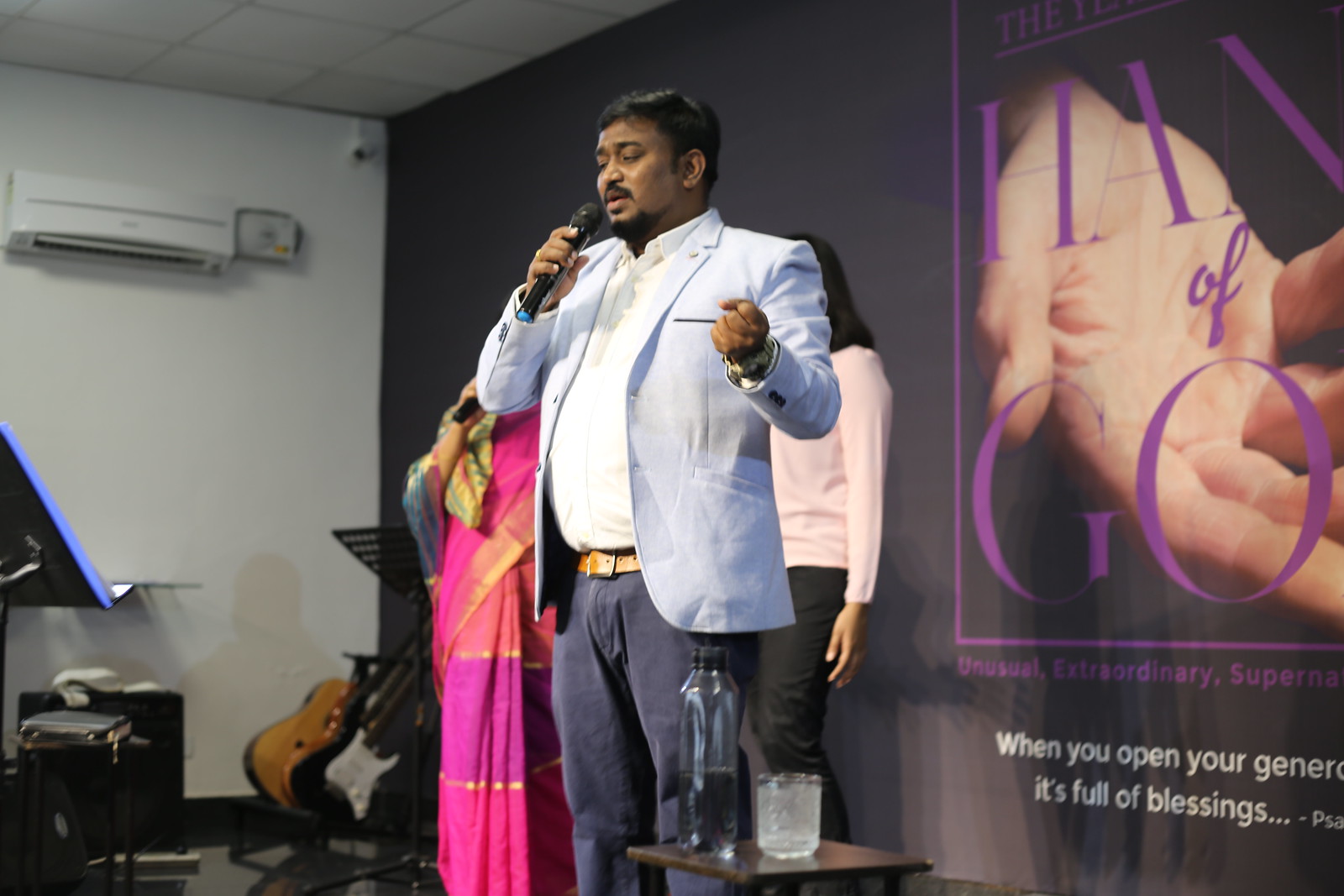The image captures an interior scene where three people are positioned on a stage, apparently engaged in singing a religious song, likely part of a Christian ceremony. At the forefront, a man with black hair and a goatee is prominently featured, clad in a light blue suit jacket, blue dress pants, and a tan belt. He holds a microphone in his right hand and has his left arm bent with a fist raised, adding an expressive touch to his performance. He appears focused, looking ahead, possibly at a stand with lyrics. To his right is a small brown table stand with a bottle of water and a glass, likely for hydration during their performance. 

To his left stands a woman in a purple and pink dress, also holding a microphone, suggesting she is singing alongside him, although her face is obscured by his body. Behind him stands another woman, identifiable by her shoulder-length hair and her attire of a white sweater and black pants. 

The backdrop features a large, black wall display with the partially visible text "Hand of God" and an image of a hand. The display also includes white text that reads "when you open your generous something it is full of blessing," referencing a Psalm, indicating the spiritual context of the scene. Additionally, two guitars are visible in the corner of the room, adding to the musical ambiance.